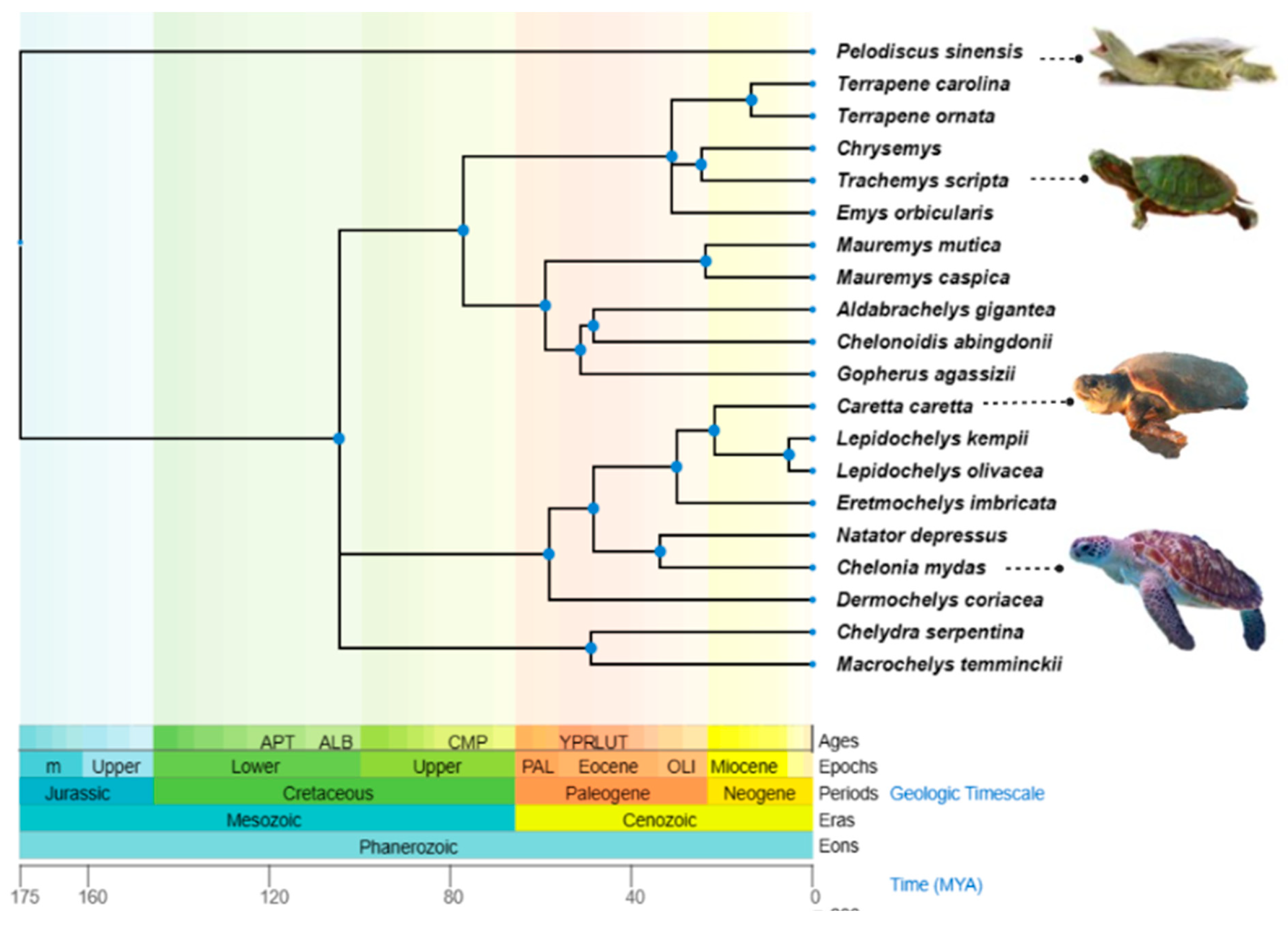This image features a horizontal flowchart that meticulously traces the evolutionary lineage of turtles from the Jurassic era onward. At the bottom, it delineates various prehistoric times, including ages, epochs, periods, eras, and eons. The chart showcases a primordial turtle from the Jurassic era, identified as the progenitor that existed through much of the Mesozoic era and approximately half of the Cretaceous period. Following this era, the evolutionary tree splits into three principal types, which continue to diversify over time, resulting in the extensive list of turtle species we recognize today. In total, the chart includes 20 different species, all named using Latin scientific terminology. Additionally, there are detailed illustrations of four distinct turtles, providing a visual representation of the evolutionary process.